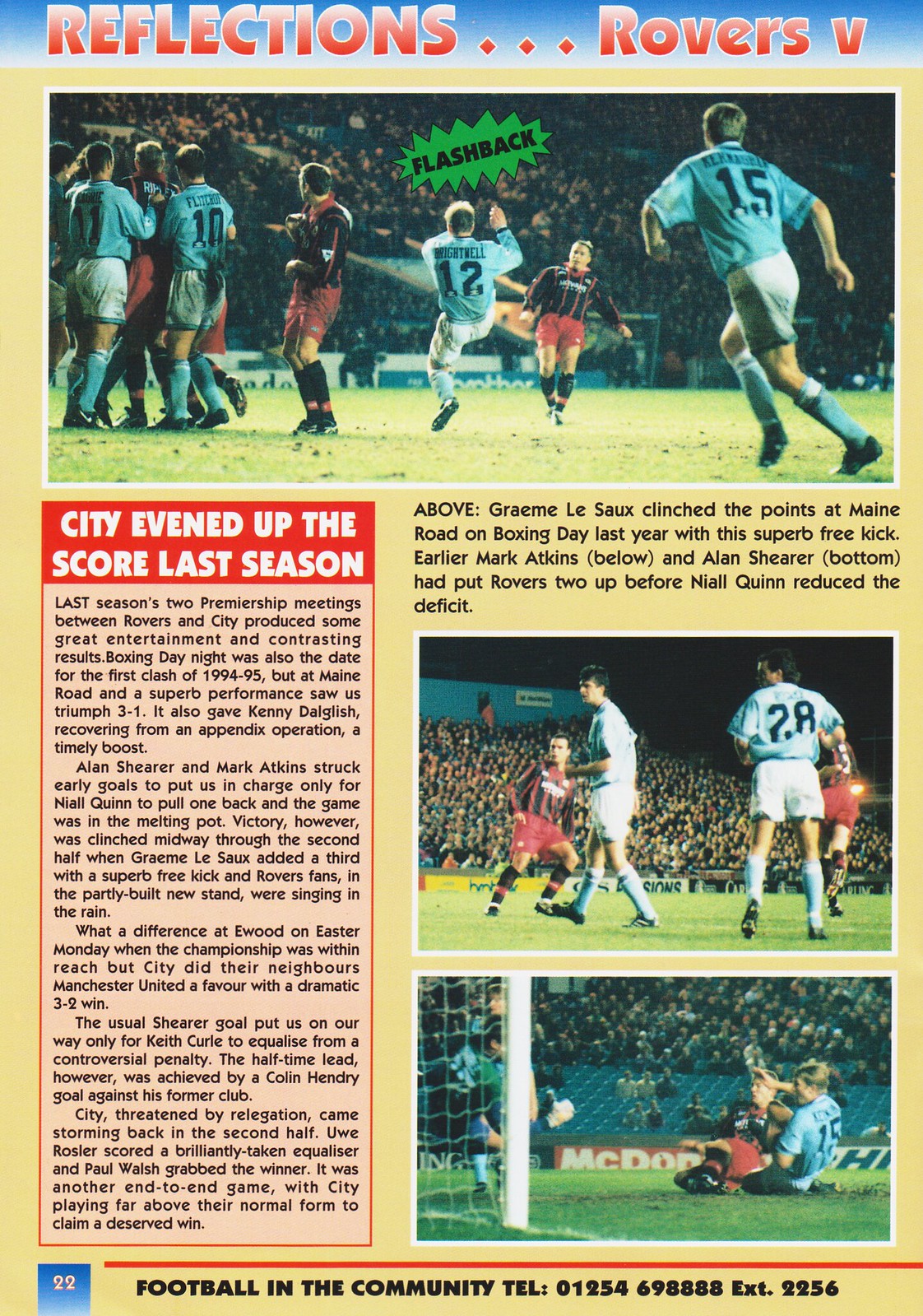The image is a detailed page from a magazine with a tan-colored background, transitioning to blue at the top. The title at the top reads "Reflections... Rovers V" in red text. Directly beneath this title is a prominent photograph featuring soccer players in red and black uniforms competing against players in teal and white uniforms on a green field. Overlaid on this picture is a green tag labeled "Flashback" in black font, indicating the nature of the content.

Central to the page on the left is a large vertical rectangle with a red-bordered pink background, and at its top, it states in dark red text, "City evened up the score last season." This section elaborates on the entertaining and contrasting outcomes of the premiership meetings between Rovers and City, highlighting key moments from matches on Boxing Day and Easter Monday in the 1994-95 season. Key points include a 3-1 victory for Rovers at Main Road, with notable performances by Alan Shearer, Mark Atkins, and Graham Le Saux. Additionally, a dramatic 3-2 win for City at Ewood on Easter Monday is recounted, marked by goals from Shearer and Colin Hendry and notable efforts by City players Keith Curle, Uwe Rösler, and Paul Walsh.

To the right of this detailed narrative is a smaller section of text in black, referring to the central photo and two smaller images below it, which showcase the game's key players and moments. The top description mentions Graham Le Saux's decisive free kick at Main Road and earlier goals by Mark Atkins and Alan Shearer. The lower descriptions correspond to pictures of players from both teams in action, with a focus on the intense gameplay and a memorable diving defense by the teal and white goaltender against a red and black attacker.

Located at the very bottom left of the page is a small blue square indicating the page number "22." Adjacent to this on the right, a red line separates a segment in black text that reads "Football in the Community" along with a contact number: Tel: 01254698888 Ext 2256.